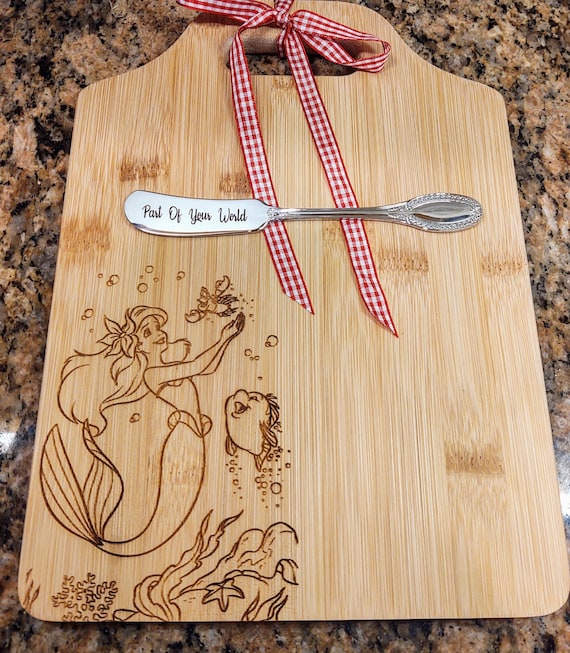The detailed close-up indoor photograph captures a light brown wooden cutting board resting on a granite countertop that features a blend of tan, black, and white hues. The rectangular cutting board, with a half-circle top and a hole for easy handling, is adorned with a white and red checkered bow tied to the top. The lower left corner of the cutting board displays an intricately carved scene from Disney’s "The Little Mermaid," showcasing Ariel holding the crab, Sebastian, with Flounder, the fish, nearby and surrounded by seaweed and underwater flora. Positioned in the middle of the board is a dull, silver spreader knife engraved with the phrase "part of your world" in cursive.